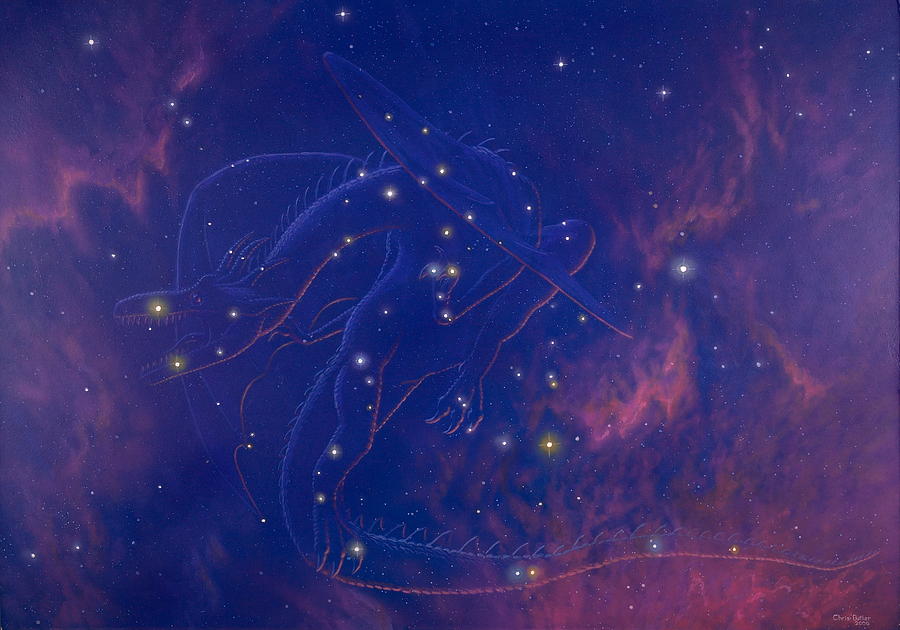In this captivating digital painting, we are treated to a mesmerizing nighttime sky in portrait mode. The deep, purplish-blue expanse is imbued with swirls of light purples and pinks, creating a visually stunning cosmos. Amidst this celestial backdrop, countless stars twinkle in hues of bright yellow and pristine white, their brilliance capturing the viewer's attention. Dominating the scene is the ethereal outline of a dragon, its nearly transparent form traced by the stars themselves. The dragon's majestic figure winds through the sky, marked by stars that delineate its open mouth, neck, body, wings, and trailing tail. The clouds, tinged with pink and lighter blue, add additional layers of depth and texture to the composition. In the bottom right corner, the name "Chris" suggests the signature of the artist, likely Chris Turner. This painting seamlessly blends the mystical allure of a constellation with the boundless imagination of mythical creatures, making it an arresting focal point within the star-studded heavens.